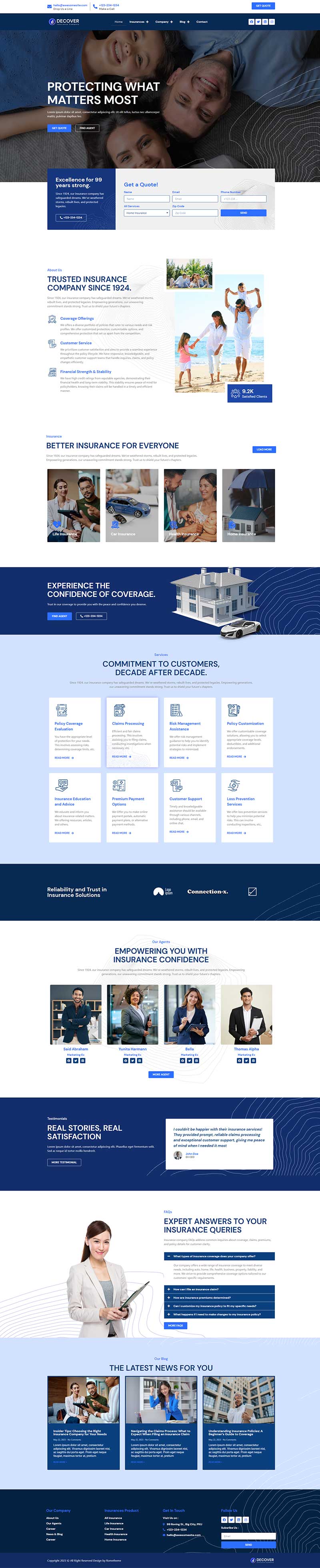A meticulously edited, elongated screenshot of an insurance company’s website is displayed in a highly minimized format, making the entire webpage viewable in a single image without the need for scrolling. The screenshot has been captured from a mobile phone, evident by its narrow width.

At the top of the page, a family photograph serves as a heartwarming backdrop. Dominating the left side is a bold, white text that reads “Protect What Matters Most.” Directly beneath this, there is an interactive box designed to collect user information for obtaining a quote. 

Further down, a thumbnail showcases a family walking along a beach, while to its right, various policy offerings are prominently listed. Below this section, a horizontal row of thumbnails visually represents diverse scenarios including people at home, a vehicle, a house, and someone typing on a computer, giving a comprehensive glimpse into the different areas the insurance covers.

A blue banner follows, featuring a vertical house icon on its right side, accompanied by a succinct paragraph to its left, likely providing additional assurances or a key message. Centrally aligned on the page are a cluster of small white boxes, each displaying different pricing options, catering to various insurance plans.

Proceeding below this price section, another horizontal row of thumbnails illustrates more real-life scenarios. Near the bottom of the webpage, an image of a doctor is flanked by detailed descriptions of medical policies, rounding out the extensive offerings provided by the insurance company.